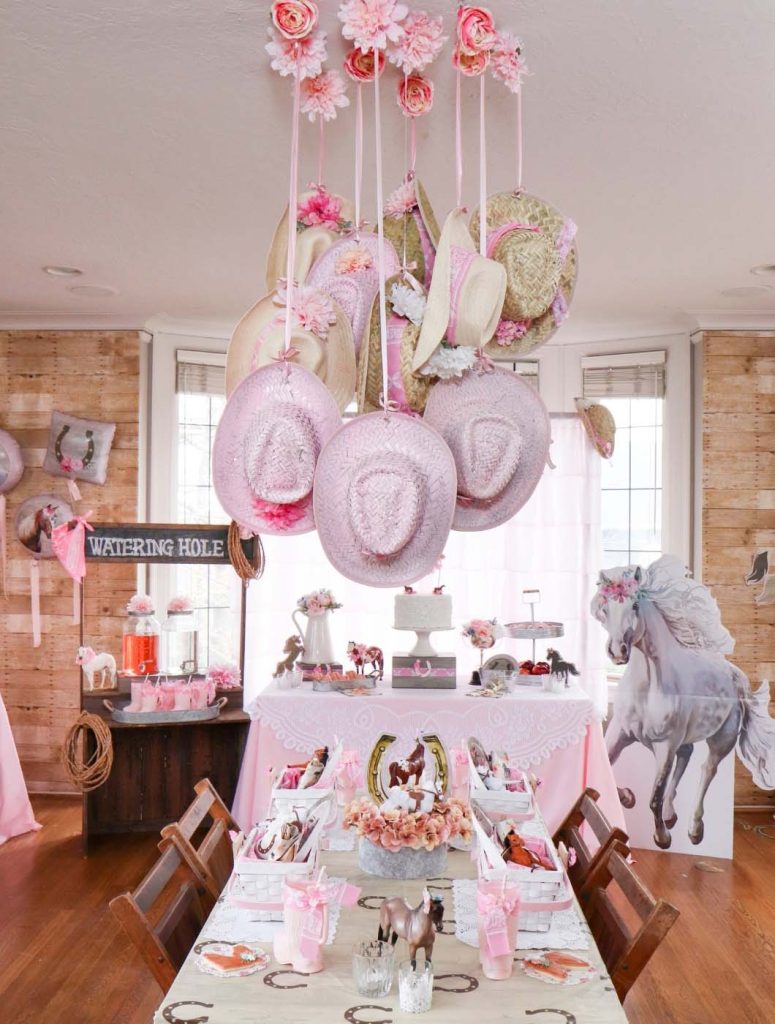This is an indoor, full-color photograph taken during the day, featuring a celebration with a rustic, horse-themed decor. The room has an off-white ceiling and brown brick walls. Hanging from the ceiling by white ribbons are an assortment of cowgirl style hats in pink and tan with pink ribbons, adding a feminine, floral touch. 

Dominating the foreground, a rectangular table draped with a horseshoe-patterned tablecloth is accompanied by four wooden chairs, each with horizontal slats on the backrest. On this table, white baskets with pink handles contain small horse figurines.

In the center of the image, a secondary table covered with a pink tablecloth and edged with a delicate pink or white doily holds several cakes. Behind it, a brown wooden stand labeled "watering hole" sits to the left. Further back, a large bay window bathed in natural light brightens the room, though the outside view is indiscernible. The window features grid-like detailing.

Adjacent to the "watering hole" stand is a decorative display with a cardboard cutout of a white horse adorned with pink flowers around its head. Overall, the scene suggests that a festive, possibly birthday-related, event is about to take place.